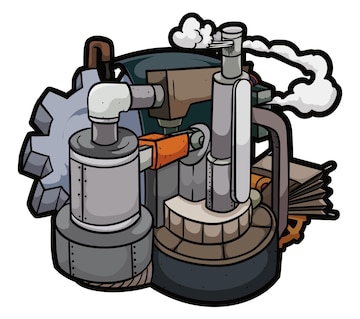The image is a detailed clip art illustration of a cartoonish, seemingly industrial machine or engine set against a white background. The machine features several cylindrical pipes and canisters in various shades of gray, brown, and dark gray, all outlined in black. Prominently, a large gray gear with pronounced teeth juts out from the left side. Linking different parts of the machine, an array of pipes extends from a central cylindrical section, connecting to a brown segment. At the top, there is a chimney-like pipe emitting white gas or smoke, suggesting some form of exhaust. On the right side, there is a brownish-beige bellows and another rust-colored gear, adding to the complex mechanical appearance. Additionally, smaller details such as bolts are visible throughout the composition, further enhancing the machinery motif.